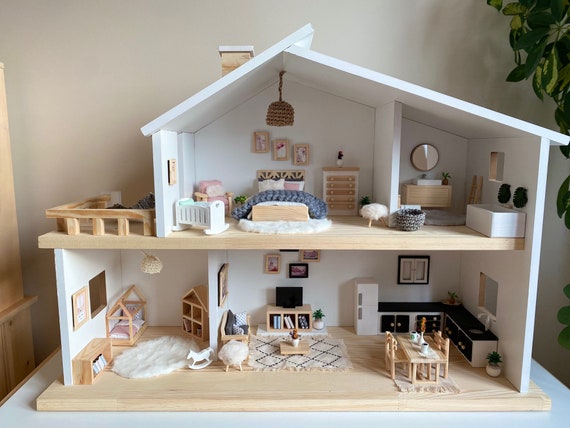This photograph captures a detailed view of a modern, white, two-story dollhouse. The ground floor features a large, open-plan living room that seamlessly connects to the kitchen and dining area. Adjacent to this space is a child’s bedroom, furnished with a small bed in the corner, a white rug, a bookcase, and a rocking horse. The upper floor includes a master bedroom at the center, which also contains a crib, flanked by a bathroom on the right. Additionally, there's a small outdoor patio on the top left, enclosed with a wooden fence. Other notable details include light wood tables, a chandelier, unique picture frames, and a miniature straw mat. The dollhouse exhibits a modern touch and is crafted from pressed wood, giving it a contemporary look. It is placed on a table against a white wall backdrop, with green grass and leaves also visible on one side.